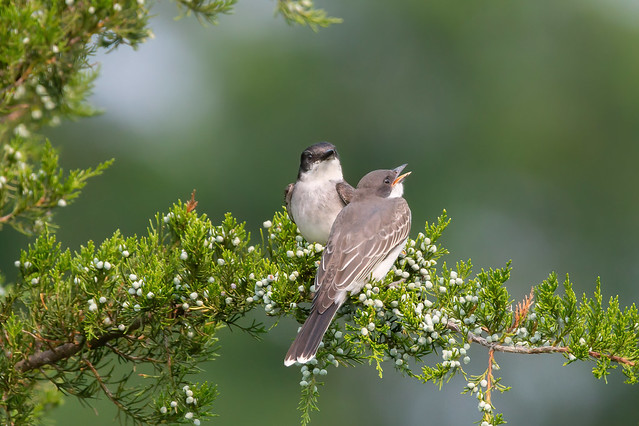This captivating nature photograph showcases two small birds perched closely together on a vibrant green branch adorned with delicate white flowers and clusters of blue-colored berries, suggestive of a juniper tree. Both birds, likely finches or a similar species, feature a striking contrast in their plumage with light gray upper bodies, darker gray tail feathers, and white underbellies. One bird, with an orange beak, faces towards the camera making it clearly visible, while the other, with a black beak, turns its head to the side, appearing to chirp. The meticulous details of their feathers are highlighted, including the streaks of white at the tips and the medium gray tones. The healthy branch includes a mix of fresh green, lightly dusted blue berries, and a few brown needles, indicating the vitality of the scene. The blurred background ensures that the viewer's focus remains solely on these charming birds, possibly singing to herald the arrival of spring. This highly detailed image vividly captures the essence of wildlife in its natural habitat.